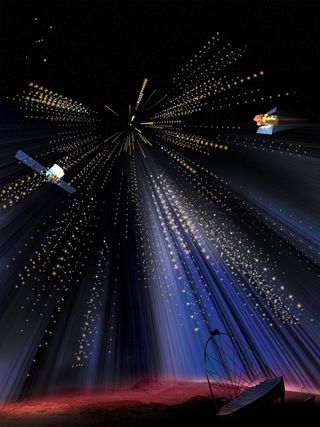The image is a vertically rectangular, multi-colored artistic representation, likely digital or print-based with no specific border or background. The scene is predominantly dark at the top, with black and bluish hues, where particles cast a bluish light downward. The lower right corner features a satellite dish with protruding spikes. In the upper right and center left regions, there are distinct yellow and white satellites with visible solar panels. White dots and lines scatter across the upper half, reminiscent of a starry sky or a time-lapse effect. The bottom section has a wavy, pink horizontal stripe and a darker area that runs along the very bottom edge, hinting at a landscape or horizon. The overall composition with its dramatic lighting and surreal elements suggests an altered or digitally manipulated image, possibly resembling a scene from a stage show or an imaginative space scene.